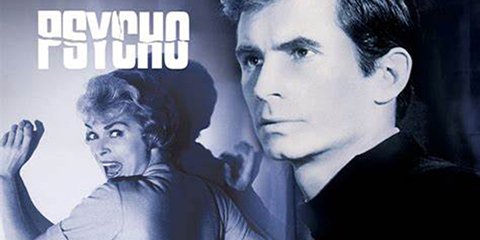This banner graphic, originating from the 1960s Alfred Hitchcock movie "Psycho," is a wide and stylized image predominantly in black and white. At the top left, the name "Psycho" is displayed in stark white, fractured block letters, giving the appearance of being slashed by a knife. Below the title, a woman is depicted with her hands pressed against a white wall, her medium-length light-colored hair framing a face frozen in a terrified scream, her eyes wide open as she looks over her shoulder. On the right side of the banner, a young, emotionless man with dark hair, presumably Norman Bates, stands in profile, wearing what resembles a black turtleneck, gazing towards the fractured text "Psycho."